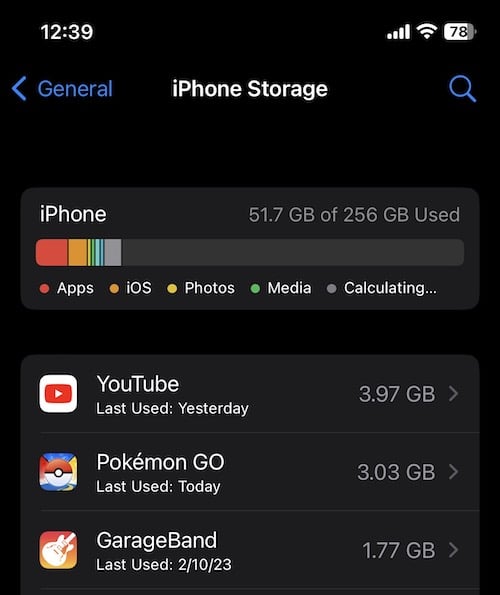This image displays a close-up of a cell phone screen's interface, capturing various details. The current time at the top reads 12:39, accompanied by indicators for battery life and Wi-Fi signal strength. On the left side, the screen shows a 'General' menu with a back arrow and 'iPhone Storage', followed by a magnifying glass icon.

Below this, there is relevant storage information: "iPhone, 51.7GB of 256GB used." A bar graph follows, color-coded in segments of red, orange, light green, dark green, blue, dark blue, and gray, representing the storage usage by categories such as apps, iOS, photos, media, and 'calculating.'

Further down, the screen lists specific apps and their storage details. It first displays YouTube, marked by a red square within a white square and a white play arrow, indicating it was last used yesterday and consumes 3.97GB of storage. Next is Pokemon Go, represented by a multicolored square, last used today, utilizing 3.03GB. Lastly, there is Garage Band, symbolized by a red and orange square with a white guitar icon, last used on February 10, 2023, taking up 1.77GB of space.